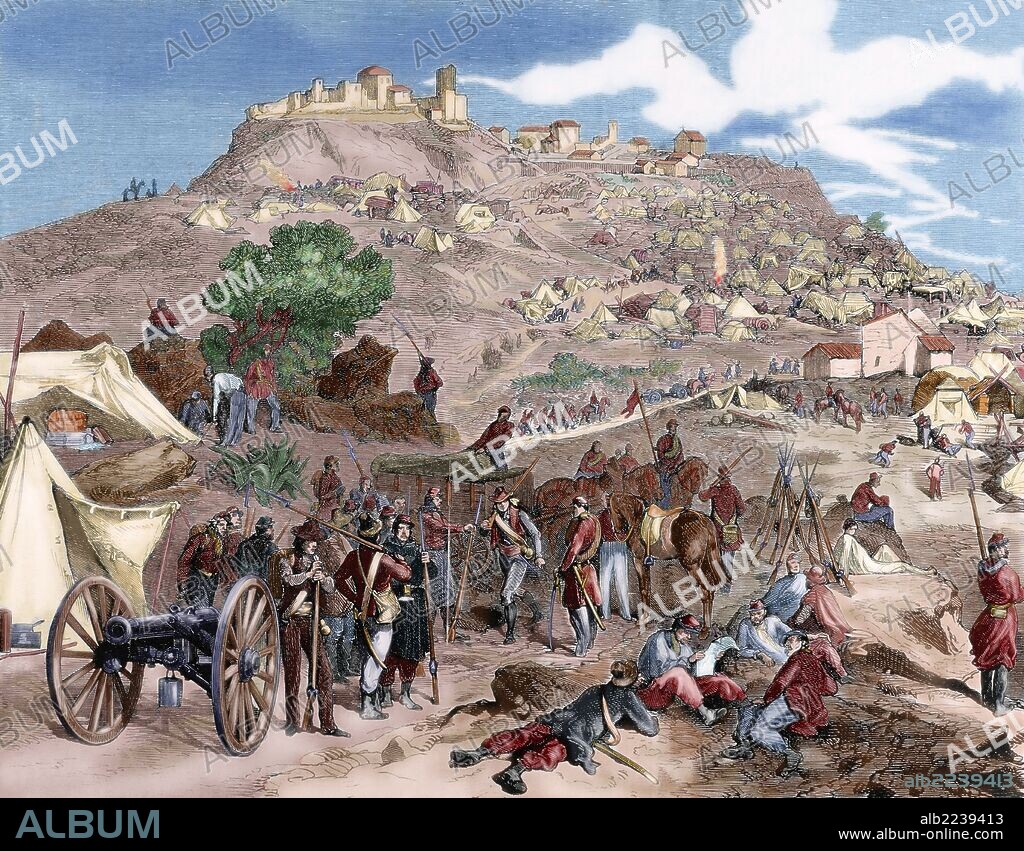This detailed painting-like illustration represents an old-fashioned battle scene set in a countryside that resembles medieval Europe. The lower part of the image prominently features raggedy tents and a cannon mounted on large wagon wheels, indicative of Old West technology. Scattered throughout are soldiers wearing red coats, 1700s-style uniforms, some standing at attention with weapons such as bayonets, while others are on the ground. To the left, several men appear to be preparing for battle alongside a mountainside dotted with a few trees and additional tents.

A winding road ascends the hill, leading to what seems to be a walled city or a substantial castle, complete with white buildings and red roofs, suggesting a strategic military target. In contrast to the historical scene, the image is overlaid with watermarks reading "ALBUM" diagonally across it. The clear blue sky with a large white cloud adds a touch of serenity to the otherwise tense atmosphere.

Further inspection of the image reveals text within a black border at the bottom. On the left, in gray font, is the word "ALBUM," while on the right, in white font, the reference number "ALB2239413" appears above the website "www.album-online.com". These details indicate the image's origin and cataloging information. Despite the watermark, the illustration captivates with its historical ambiance and intricate detail, from the military figures to the imposing castle in the distance.